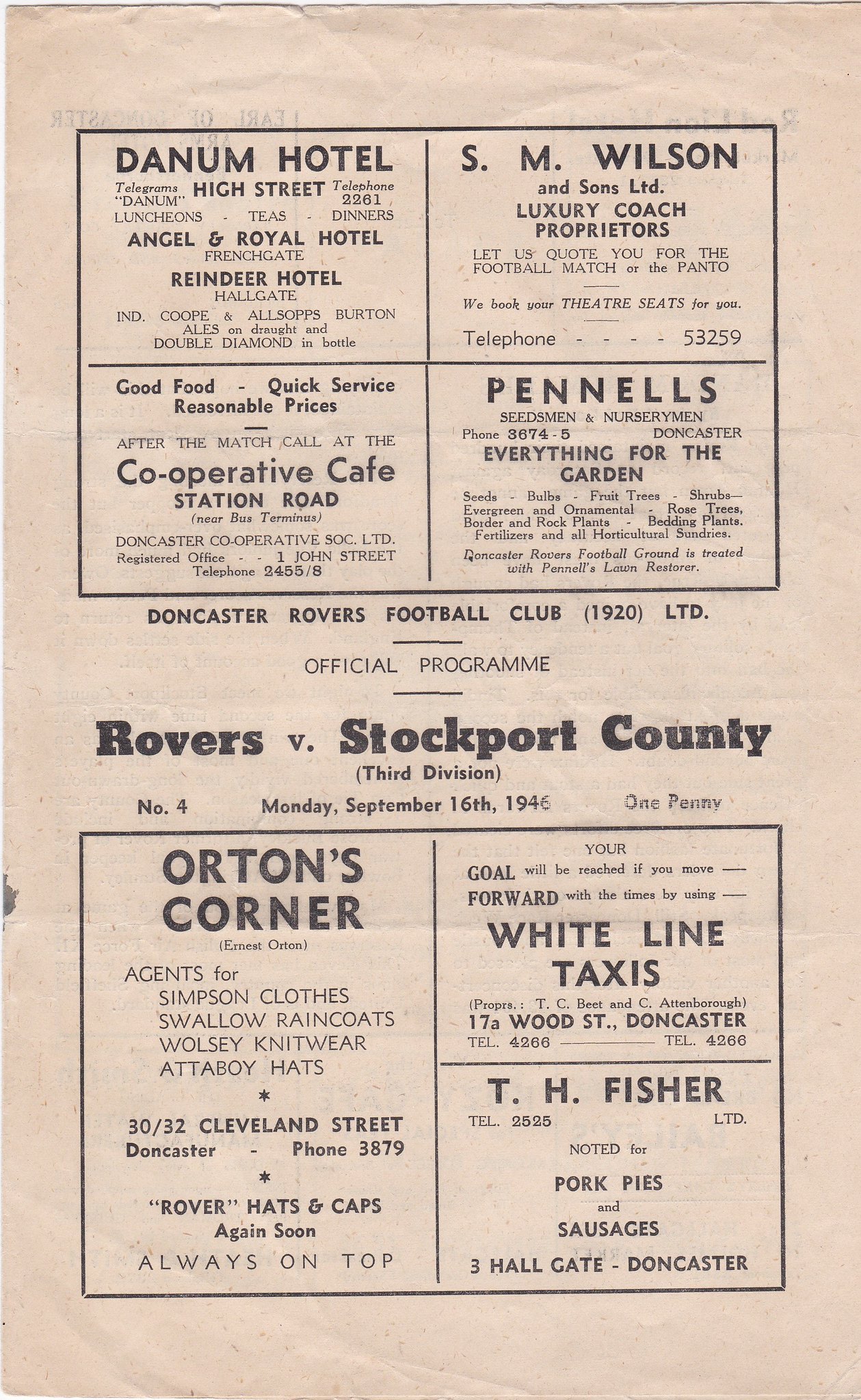An antique football program from 1920, showcasing the Third Division match between Doncaster Rovers and Stockport County on Monday, September 16, 1920. This official program, bearing the text "Doncaster Rovers Football Club 1920 LTD," features various advertisements around the central match details. At the top left is an ad for Danum Hotel on High Street, while to the top right, S.M. Wilson and Sons Limited promote their luxury coach services. The ad below that is for Cooperative Cafe on Station Road with the tagline "Good Food, Quick Service, Reasonable Prices," and further down, Pinnell's offers "Everything for the garden." The bottom section of the program includes more advertisements; on the left, Orton's Corner, and to the right, White Lion Taxis above an ad for T.H. Fisher Pork Pies and Sausages. The program is printed in black text on cream-colored, slightly wrinkled paper, with each advertisement occupying distinct sections within the layout.